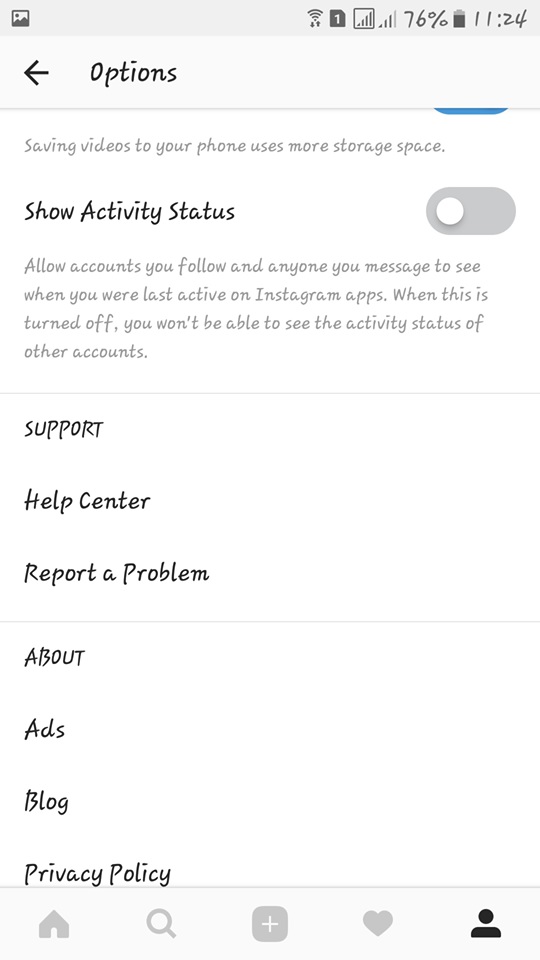The screenshot displays a cell phone screen with various interface elements and settings, likely from an app's settings or information section.

### Top Banner
- **Background Color:** Light gray
- **Left Corner:** 
  - **Icon:** A square containing a circle at the top left corner with what appears to be mountains at the bottom.
- **Right Corner:**
  - **Icons and Indicators:**
    - Wi-Fi signal icon
    - SIM card icon with the number "1" inside
    - Square icon with a cell signal icon inside
    - Cell signal icon next to it
    - Battery icon displaying "76%"
    - Current time: "11:24"

### Main Content Area
- **First Section:**
  - **Navigation:** Left-pointing arrow icon
  - **Text:** "Options" (capitalized "O")

- **Divider Line**

- **Second Section:**
  - **Text:** "Saving videos to your phone uses more storage space."

- **Third Section:**
  - **Title:** "Show Activity Status" (standard case)
  - **Description:** Allows accounts you follow and message to see when you were last active on Instagram apps. It notes that if this setting is turned off, you won't be able to see the activity status of others.

### Divider Line

- **Fourth Section:**
  - **Subheadings and Options:**
    - "SUPPORT" (all caps)
    - "Help Center" (capitalized "H" and "C")
    - "Report a Problem" (capitalized "R" and "P")

- **Fifth Section:**
  - **Subheadings and Options:**
    - "ABOUT" (all caps)
    - "Add" (capitalized "A")
    - "Log"
    - "Privacy Policy" (capitalized "P" and "P")

This detailed description provides a comprehensive understanding of the various elements displayed on the cell phone screenshot, including navigation icons, status indicators, and text options for user settings and support.